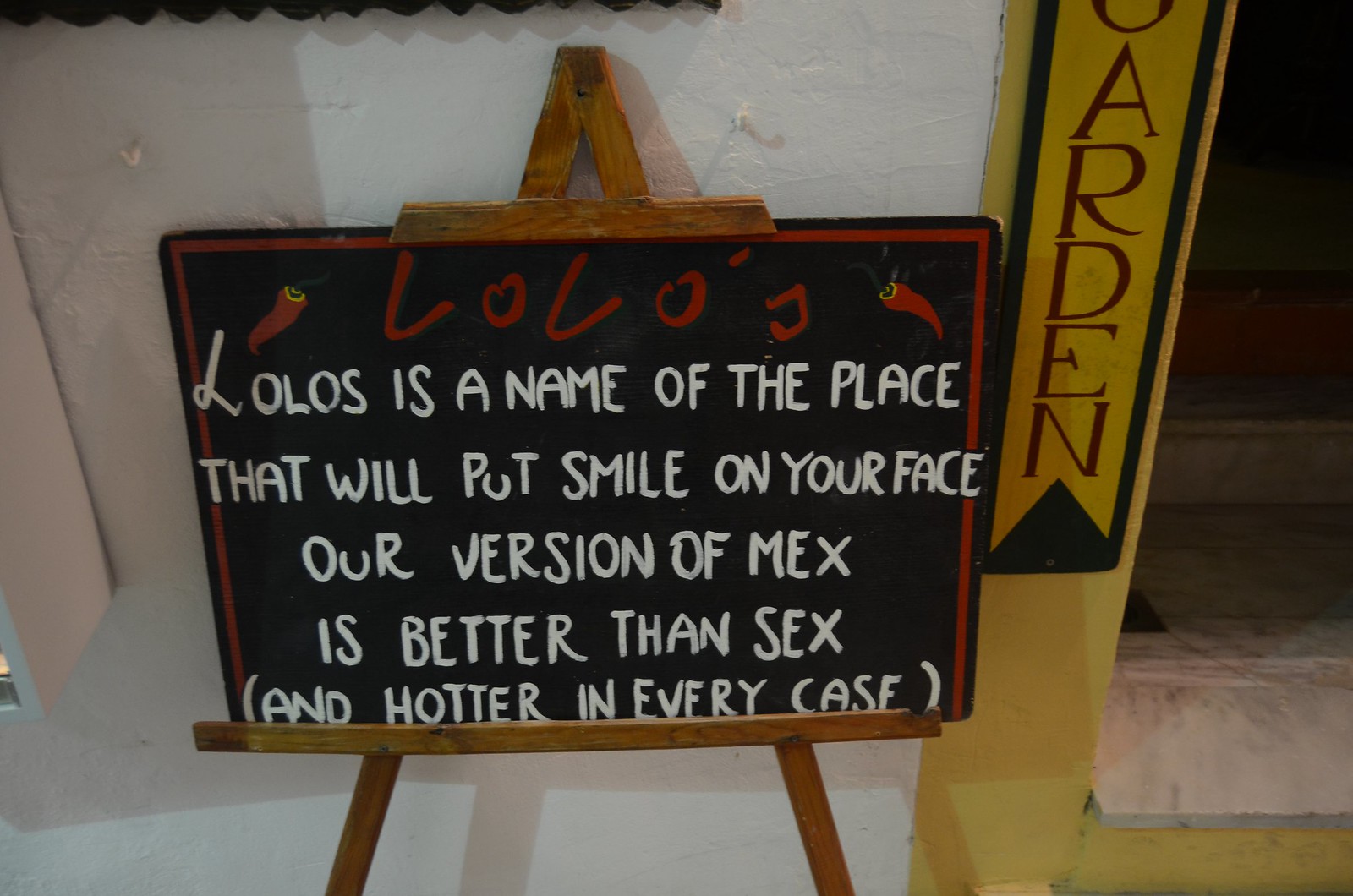In this photograph, a wooden easel stands against a white wall, supporting a black chalkboard-style sign with a red border. The top of the sign features the name "Lolo's" in red letters, flanked by red chili pepper images on each side. Below that, in white print, it reads: "Lolo's is the name of the place," followed by the lines "we'll put a smile on your face," "our version of Mex," "is better than sex," and, in parentheses, "and hotter in every case." To the right of the easel, a yellow doorway is visible with the word "garden" painted vertically in red, although the 'G' is cut off at the top of the image. A yellow border runs along the bottom of the doorway, adding a splash of color to the scene.